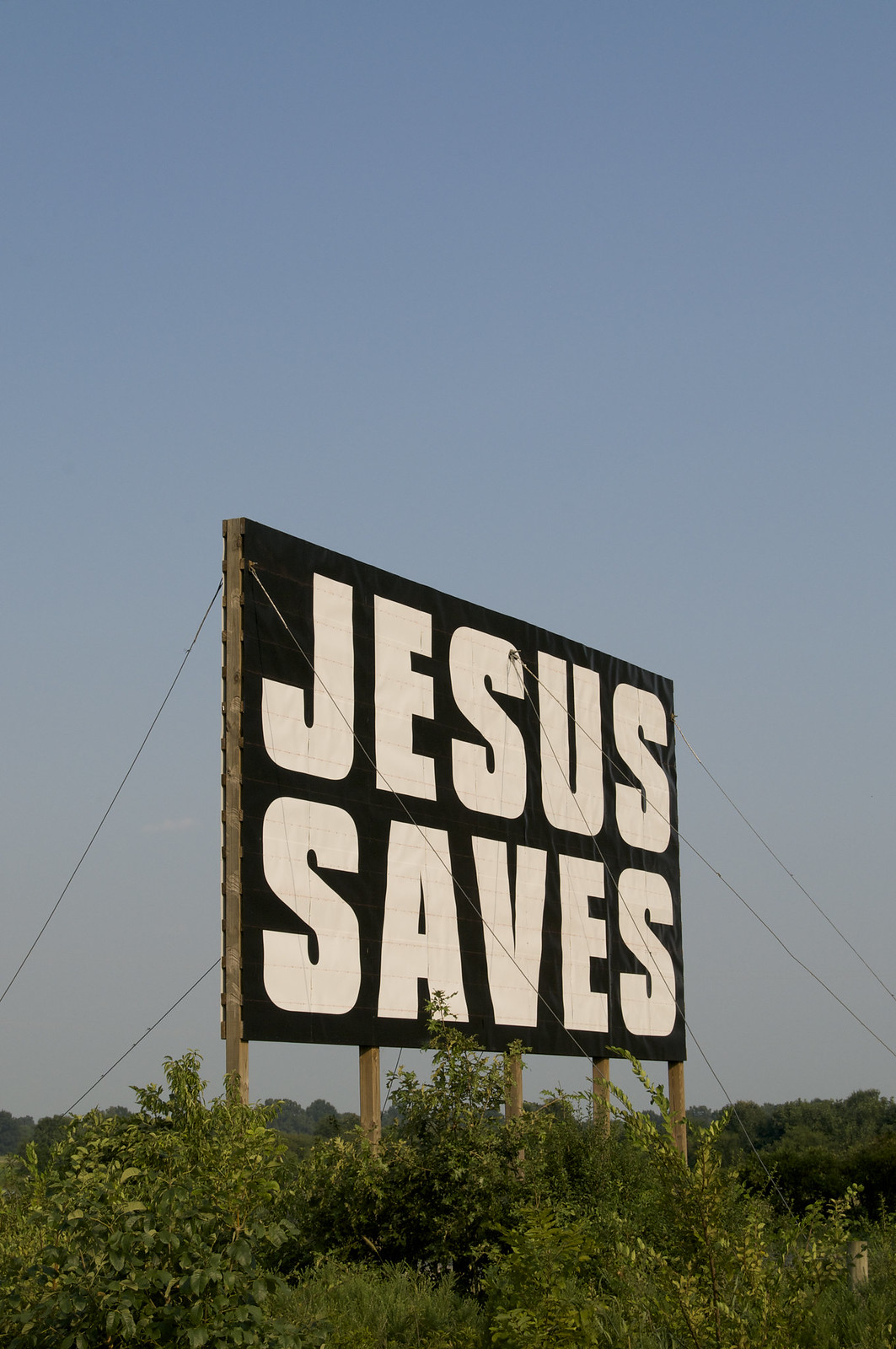This image captures a wooden billboard prominently displaying the message "JESUS SAVES" in bold, white block letters against a stark black background. The structure of the billboard is supported by several sturdy wooden beams, specifically 2x4 or 2x6 planks, with a total of five beams visible beneath it. The construction is further stabilized by four cables securing one side, and what appears to be three visible cables on the opposite side, suggesting a likely fourth cable out of view. The base of the billboard is surrounded by a mix of tall and short weeds, indicating an unkempt area beneath it. Overhead, the sky stretches out a clear, serene blue with no visible objects or obstructions in the background, creating a striking contrast to the bold, simplistic message of the sign.